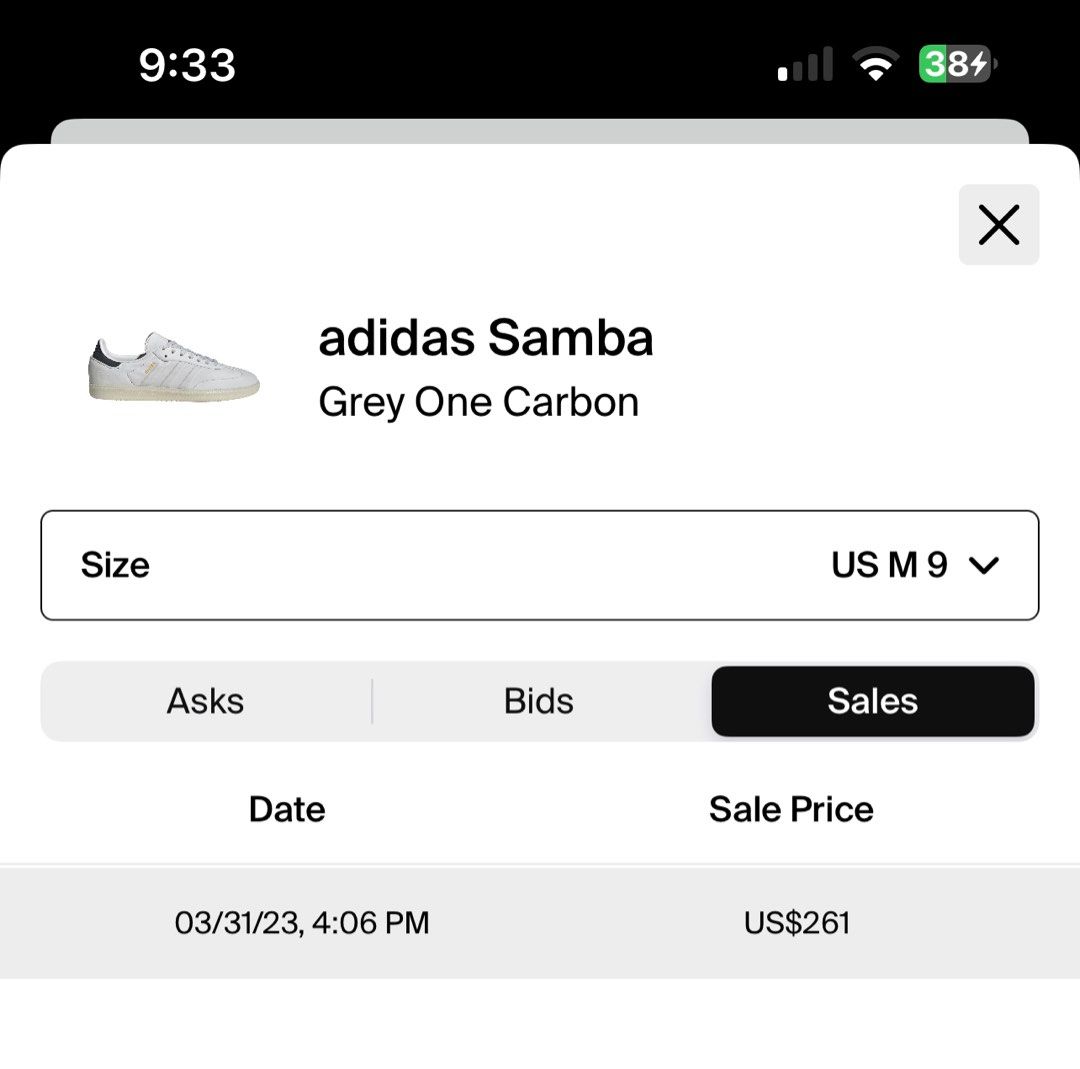A screenshot displays a mobile web store's purchase or order screen. The black border at the top interface indicates its operation on a mobile device, as shown by the time, battery life, and other standard info indicators. The top bar reads "9:33" in white font for the time, shows a 38% battery life represented by a green icon in the upper right corner, and indicates a Wi-Fi strength of 2 out of 3 bars alongside 1 out of 4 bars for mobile data connectivity.

The main content is presented in a white pop-up menu that can be closed by tapping the 'X' in the upper right-hand corner. Dominating the display is an image of a white-colored sneaker, identified as "Adidas Samba Gray 1 Carbon." Below the image, the size is listed as "Size US M9" with an accompanying drop-down arrow, suggesting size options. Further down, the interface lists details under section headers such as "Asks," "Bids," "Sales," "Date," and "Sale Price." Specifically, in the "Date" column, the entry reads "3/31/23 at 4:06 PM.” In the "Sale Price" column, the cost is noted as "US $2.61."